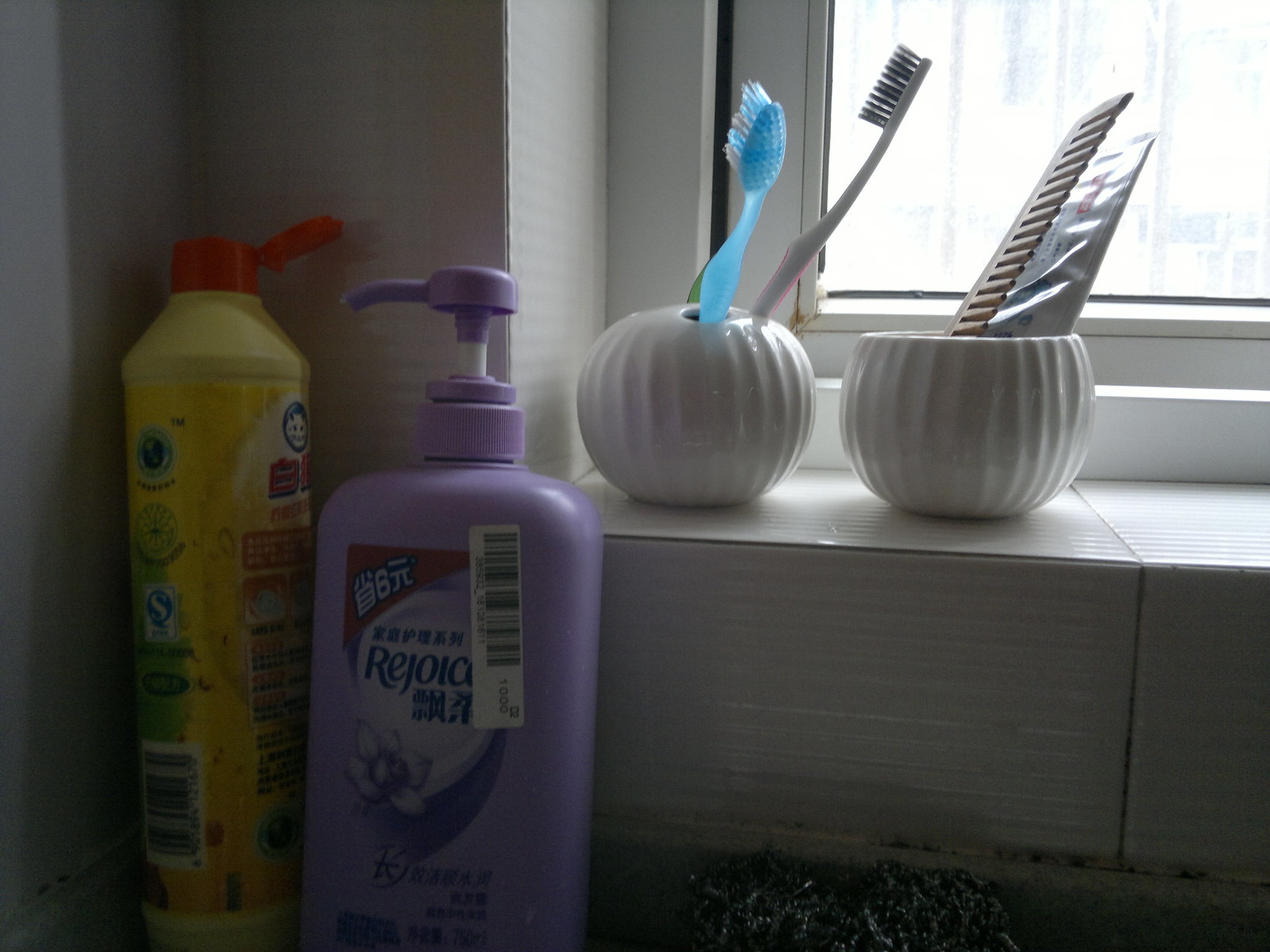This photograph captures a dimly lit bathroom corner with a white-tiled windowsill that holds a collection of toiletries. In the upper right of the image, a window allows bright sunlight to flood into the otherwise dark space. The windowsill itself is adorned with two circular white containers featuring linear patterns. One container holds a blue toothbrush and a white toothbrush with black bristles, while the other contains an upside-down tube of toothpaste and a light brown comb. Below the windowsill, on the counter, are two plastic bottles: a purple hand lotion bottle adorned with red and dark purple accents alongside the word "rejoice" and some Asian lettering, and a yellow bottle with a red open cap. The detailed arrangement of everyday items against the backdrop of sunlight pouring through the window adds a warm, lived-in feel to this intimate space.